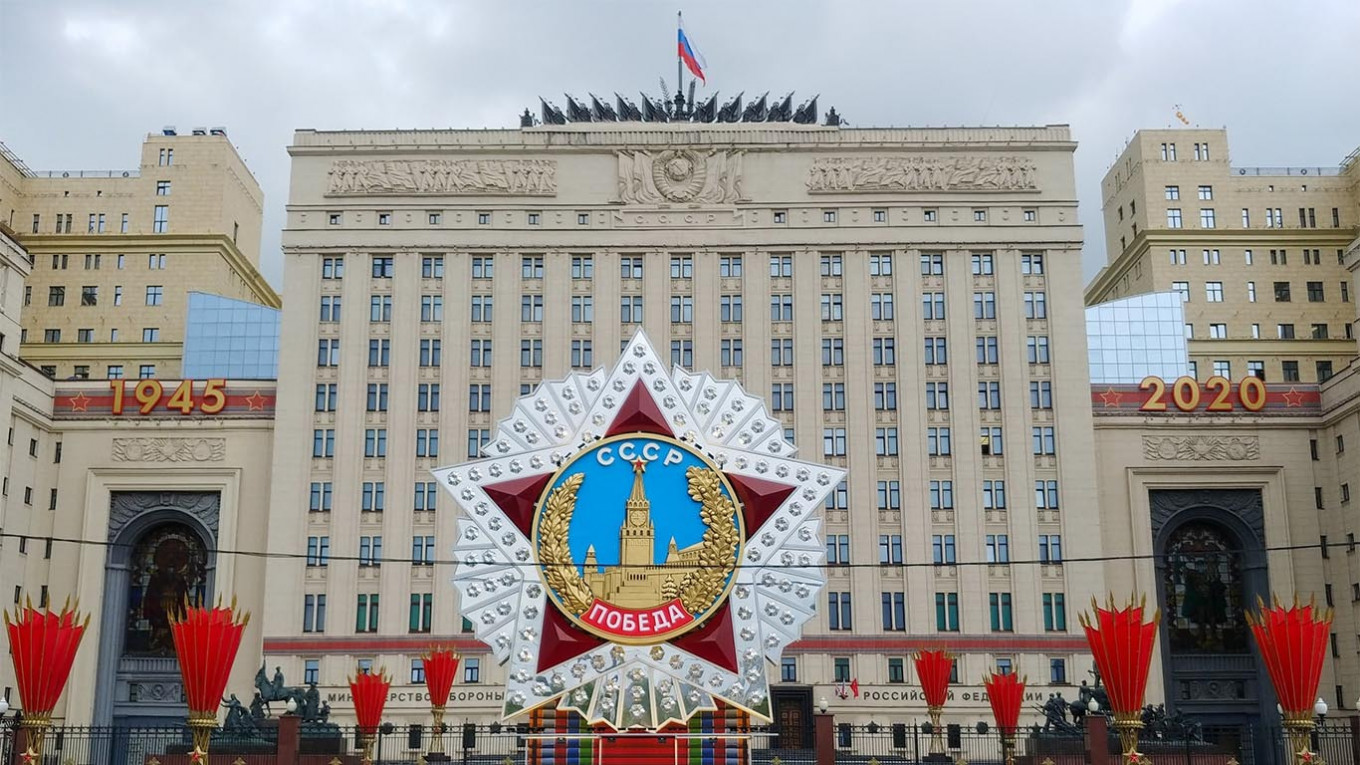The photograph captures an imposing government building in Russia, distinguished by its towering rectangular form that spans at least ten stories. The facade is clad in gray stone with numerous windows punctuating its surface. The structure boasts two wings extending to the left and right, each marked by an alcove; the left wing bears the year "1945" and the right wing displays "2020." This suggests a commemorative theme, possibly celebrating Soviet and post-Soviet history. At the pinnacle of the building, the Russian flag flutters against a backdrop of a cloudy sky.

Prominently situated in the foreground is a large, eye-catching emblem. Central to this emblem is a gold-toned depiction of a building with a spire, flanked by wreaths on either side. The emblem is set within a red star, encircled by riveted silver bars. Above the central image, the initials "CCCP" are inscribed, while Russian text, difficult to read, stretches along a curved red banner at the base of the circle.

Adding to the visual complexity, numerous red, inverted cone-like decorations, resembling upside-down umbrellas or perhaps stylized fireworks, line the area just outside a fence that delineates the building’s grounds from the sidewalk. In the background, two additional tall buildings hint at the scale of the surrounding urban landscape. The entire scene is set under a gray, overcast sky, amplifying the solemn grandeur of the setting.